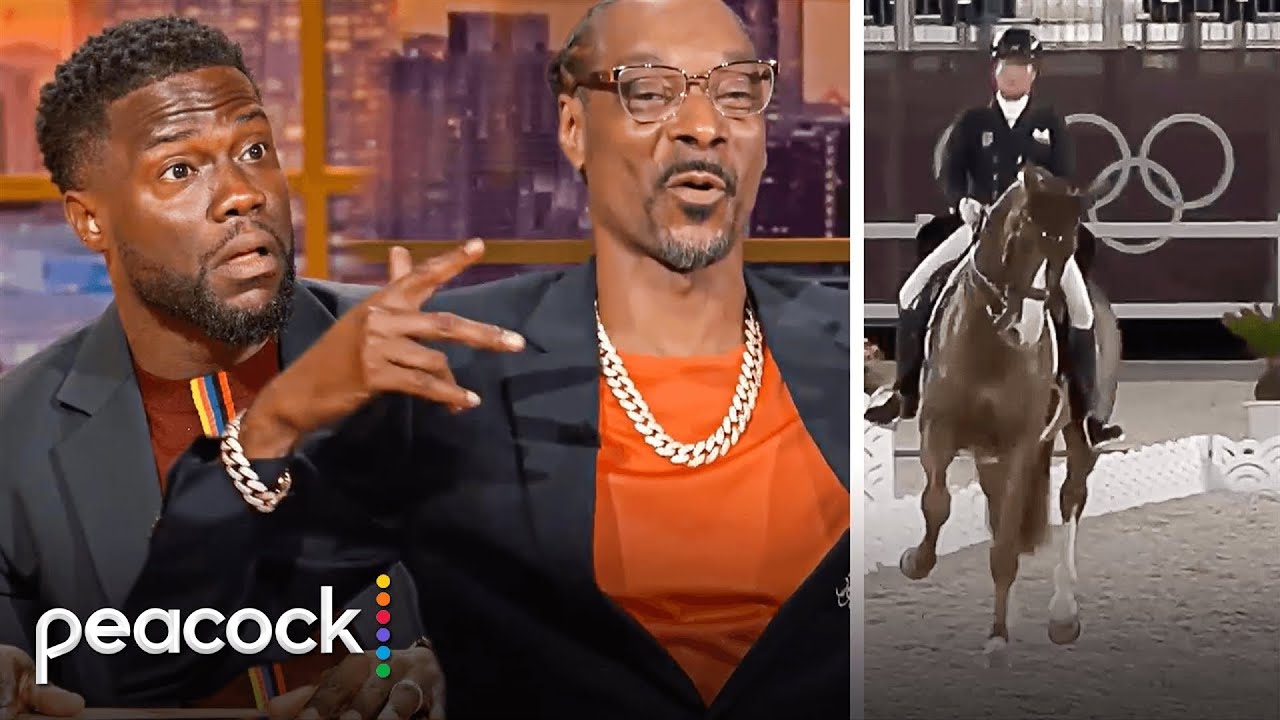In the left part of the two-part image, comedians Kevin Hart and rapper Snoop Dogg appear on what looks like a talk show set, likely from the Peacock network, as indicated by the logo in the lower left corner. Kevin Hart, identifiable by his short black hair, goatee, and wide-eyed expression suggesting surprise or agitation, is wearing a gray suit jacket with a distinctive shirt featuring an African-colored stripe. Next to him, Snoop Dogg, recognizable by his dreads pulled back, eyeglasses, and chain necklace, sports a black suit jacket over an orange shirt. The background hints at a late-night talk show setting with wooden panels visible to the right.

On the right side of the image, there's a dynamic scene of a jockey riding a galloping brown horse with a white patch on its nose. The jockey, dressed in a black jacket, white pants, and a black hat resembling a state trooper's hat, rides energetically against a backdrop featuring a low white fence and what appears to be Olympic symbols on a distant wall. The ground beneath the horse is sandy or gray dirt.